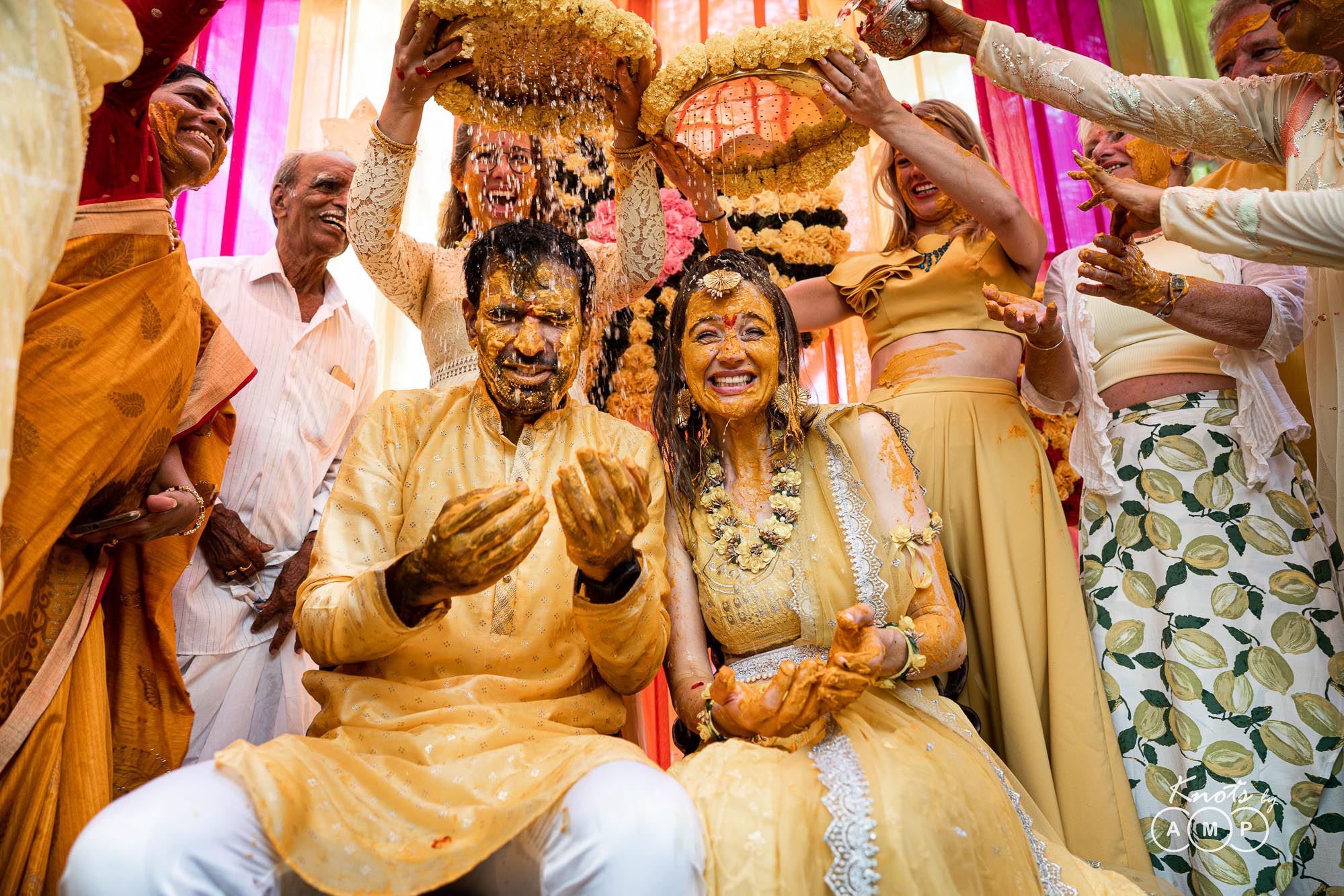The image captures a joyous moment from what appears to be a traditional Indian wedding ceremony. The newlywed couple, dressed in traditional attire, sits amid a colorful and vibrant setting. The bride, adorned with flowers around her neck, wears a beautiful outfit complemented by the groom's white pants and a traditional Indian tunic. Their hands are extended as friends and relatives, forming a semicircle around them, engage in a ritual of pouring a turmeric-like paste through a mesh screen adorned with flowers. This paste, golden in color, drips down, symbolically bathing the couple in blessings. The women attending are dressed in elegant midriff tops and flowing skirts, with some in traditional sarees, while the men wear ornate tunics paired with white slacks. The backdrop is a burst of colors, predominantly pink and gold, adorned with flowers and bright lights, adding to the celebratory atmosphere. The couple's faces glow with happiness as they partake in this sacred and age-old tradition.